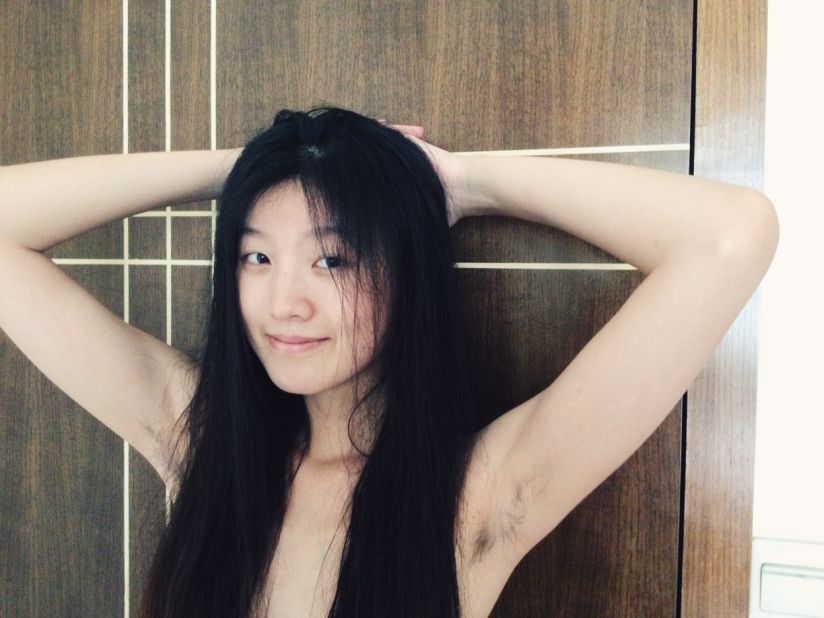In the image, an Asian woman with long, straight black hair stands confidently indoors, in front of a brown wooden wall that features a crisscross pattern with inlaid white wood. She has pale skin and appears to be topless, though her chest is covered by her hair, and the picture only goes down to her chest. The woman is posing with her arms raised behind her head, fingers locked, and she has noticeable armpit hair, which is also black. Her face is free of makeup, highlighting her natural beauty, and she has a smile on her lips. The description of her hair mentions it being stringy and dry, adding texture to the detailed portrayal.